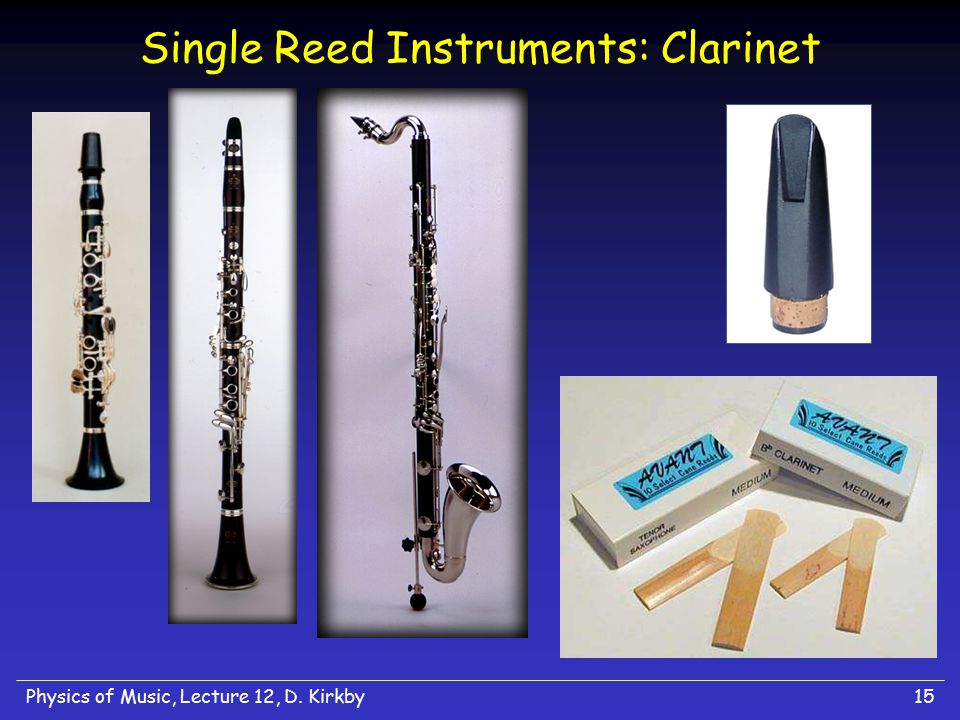The image depicts a detailed informational slide from a college course presentation titled "Physics of Music, Lecture 12, D. Kirkby." The main focus of the slide is on single reed instruments, particularly the clarinet. The slide features three black and silver clarinets vertically arranged on the left side. In the top right, there is a clarinet mouthpiece, while the bottom right displays several reeds next to their boxes labeled "Clarinet, Medium, No. 15." The background of the slide has shades of blue and purple, with text in yellow and white. The slide's style is characteristic of a PowerPoint presentation used for educational purposes, emphasizing the physics of music related to single reed instruments.